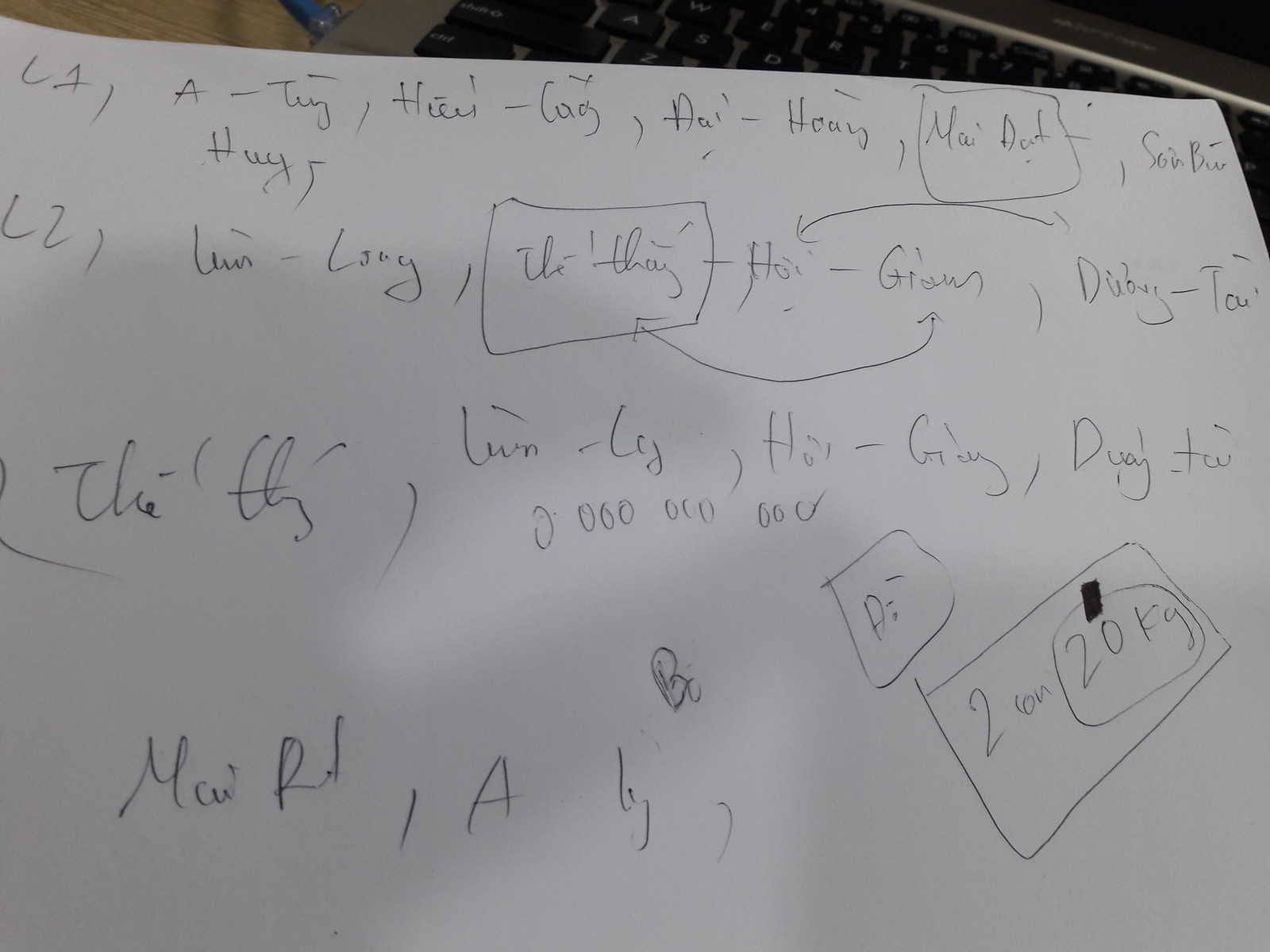This is an image of a white piece of paper that appears to be somebody's homework, written in a language other than English. The text is structured into two main sections labeled "L1" and "L2".

On the left side, under "L1," there is a list of words separated by commas, with one of the words highlighted with a box around it. The words are patterned, featuring a sequence of three letters followed by a dash and then more letters. This pattern repeats throughout the "L1" section.

Below this, the "L2" section follows a similar format, with three-letter sequences separated by dashes and commas. This section includes a boxed area with an arrow, suggesting that the order of the words within the box has been corrected. 

At the bottom right corner of the page, there is a diagonal box containing the letters "AI." Below this, there is a larger rectangle that contains the text "2 on" or possibly "ton." Inside this rectangle, an inner oval shape holds the inscription "20 kilograms."